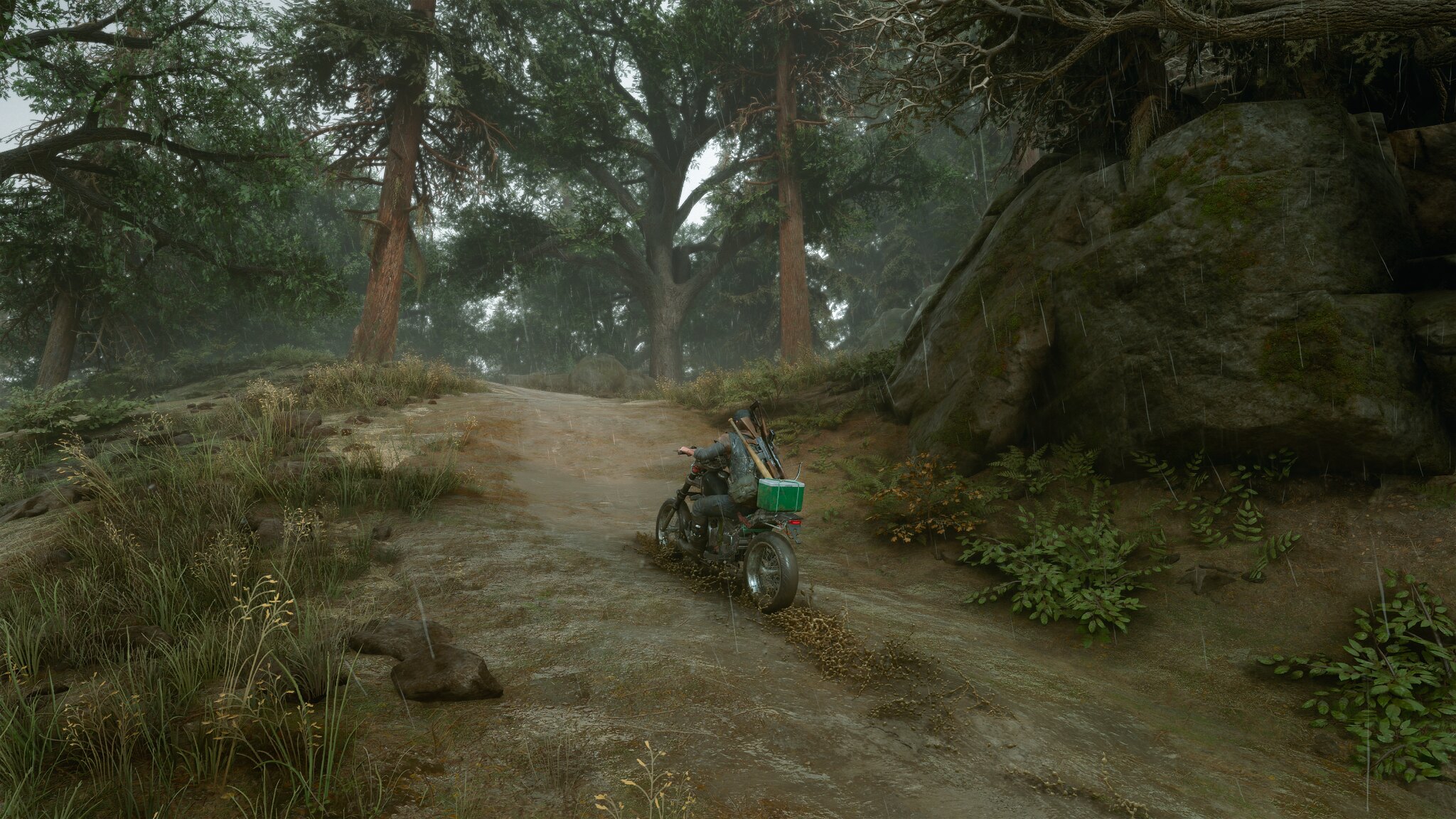In this color screenshot from the video game "Days Gone," the protagonist, Deacon, is seen riding a motorcycle up a steep, brown dirt hill. With his back to the camera, Deacon is clad in a dark, long-sleeved jacket and has a messenger bag slung over his left shoulder. His rugged appearance is heightened by the numerous items strapped to his back, including a baseball bat and two rifles. A green cooler is securely fastened to the rear of the motorcycle. The tires of the motorcycle are kicking up a significant amount of mud as Deacon navigates through the rain-soaked terrain. The environment around him is lush with greenery, accentuated by a towering rock formation on the right side of the image. Thin, white vertical lines indicating rain streak across the scene, adding to the immersive and gritty atmosphere of the game.